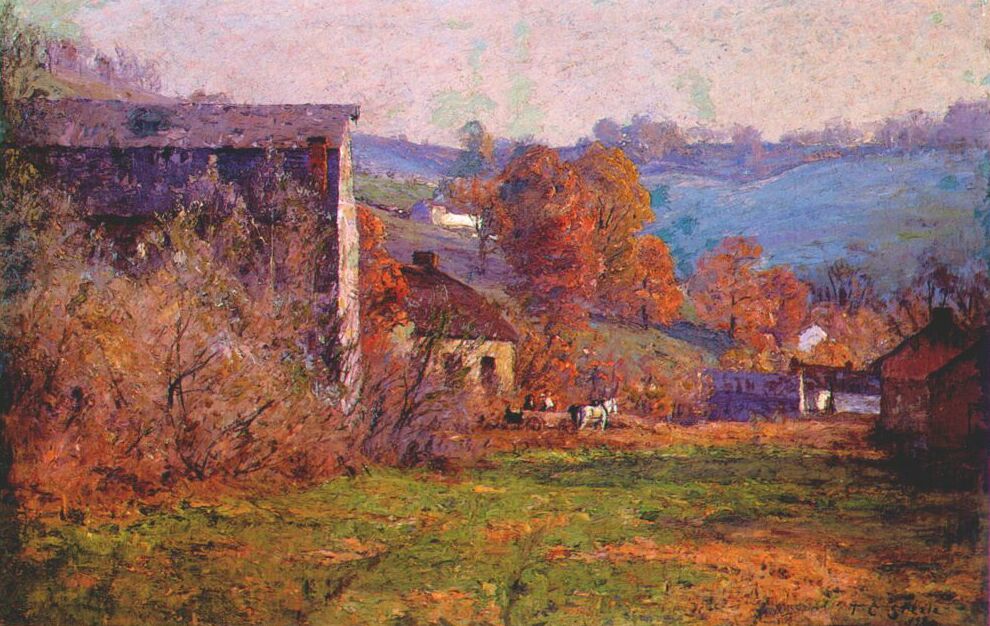This captivating impressionist painting depicts a vibrant fall scene in a sprawling rural village. Dominating the foreground is a large, lush field blanketed with a mix of green and orange leaves, signifying autumn. Brown leaves cascade gently from trees, creating a picturesque landscape. On the left, there's a rustic farmhouse with a purplish-red roof and a distinctive red chimney, nestled amid dense shrubs. In the distance, clusters of houses and log cabins with similar red roofs dot the landscape, each adding a touch of charm to the serene setting.

A white horse with a brown tail stands prominently with a saddle on its back, near which two figures are visible, possibly sitting by a trough or hedge, enhancing the painting's pastoral feel. To the right of the figures is a small utility cabin, and farther to the left, a large barn stands tall. Towards the very back of the scene, a mountain range rises majestically under a grayish to purplish sky streaked with hints of orange light. The sky's soft, fuzzy texture might suggest an aged photograph effect, adding depth to the scene. In the lower right corner of the painting, the artist's signature, T.C. Stevie, is etched in black, grounding this evocative piece in personal authenticity.